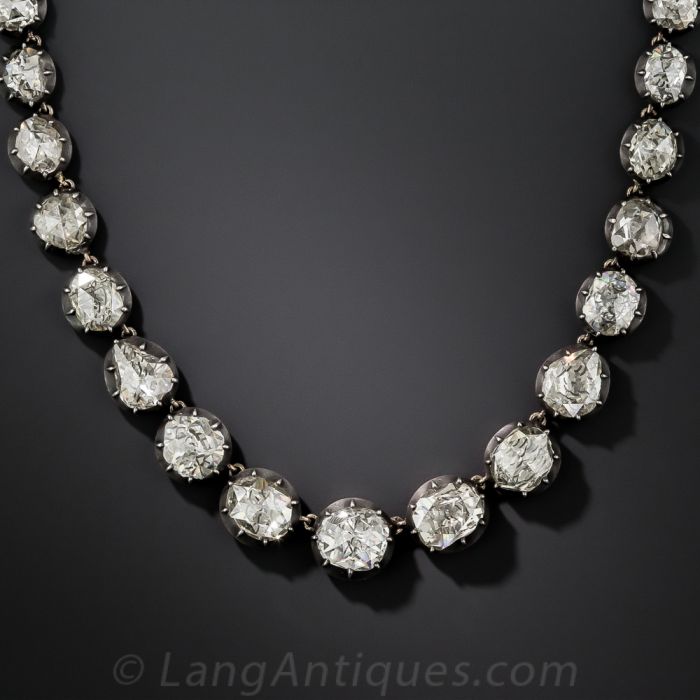This is a detailed close-up photograph of an elegant necklace, displayed against a dark gray or black background with a watermark at the bottom reading "LangAntiques.com." The necklace features individually set stones—likely diamonds, though they could be high-quality imitations such as rhinestones or cubic zirconia—each situated within silver or possibly sterling silver settings, which is unusual as they do not appear to be gold. The design is akin to a tennis necklace, suggesting a continuous line of stones. The diamonds or stones progressively decrease in size from the center, where the largest diamond is prominently placed to rest between the collarbones, down to the smaller ones toward the clasp. The settings encase each stone so that only the top is visible, creating a seamless look of brilliance and coherence. Although we see only a portion of the necklace and cannot ascertain the length or the fasteners, it is unmistakably a beautiful and meticulously crafted piece, indicative of vintage jewelry offered by Lang Antiques.